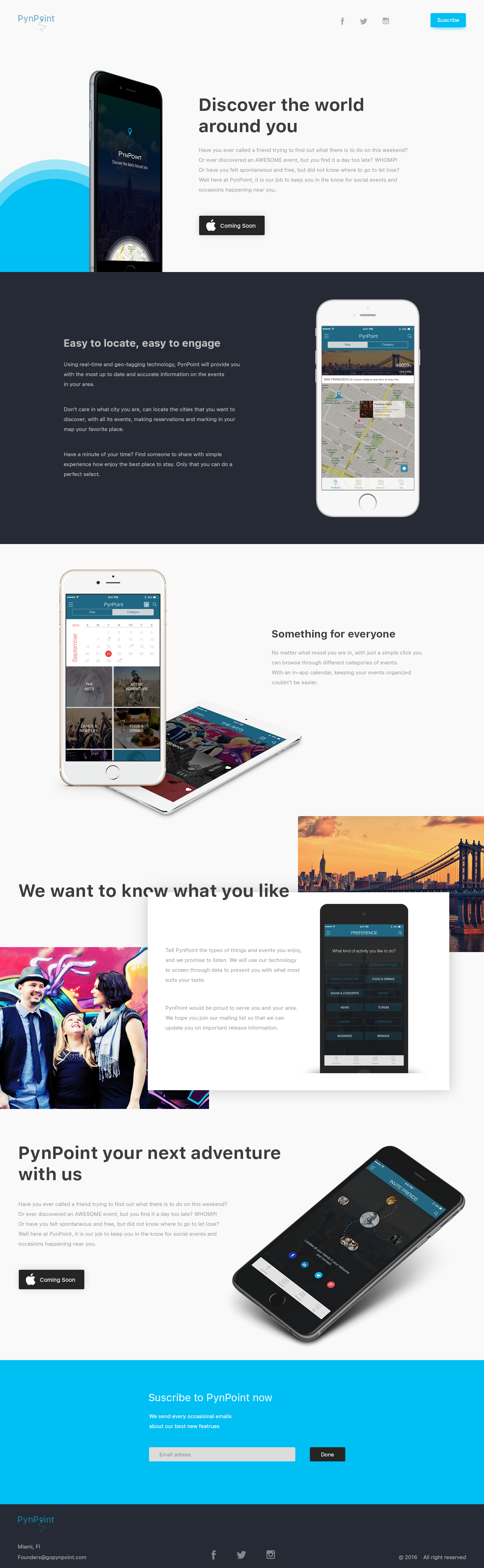This distorted advertisement showcases the upcoming launch of the Pinpoint application, an app devised to help users discover local events and activities. At the top, the ad features an image of a smartphone displaying the Pinpoint logo along with the tagline, "Discover the world around you."

The ad's first section addresses common frustrations of missing out on local events. It asks whether you've ever called a friend to find weekend plans or stumbled upon an event too late. Pinpoint aims to eliminate such issues by keeping you informed of social events and occasions nearby. This section is followed by the Apple icon with the note "Coming Soon," indicating that the iPhone app will be available shortly.

Below, another phone screen image illustrates the Pinpoint app in use, featuring a map interface under a banner with menu and category options. The app shows various interactive icons categorized under interests such as arts, active adventures, nightlife, and food and drinks.

The next segment of the ad emphasizes personalization, asking users about their preferences. The phone screen example lists activities like arts, active adventures, nightlife, food and drinks, shows, concerts, news, and tourism. Although some text is distorted, it suggests a tailored user experience based on individual interests.

The final section encourages users to "Pinpoint your next adventure with us." It displays another phone screen showing an "Invite Friends" feature, symbolized by icons connected to depict user relationships. At the bottom, a call-to-action invites users to subscribe to Pinpoint. There is an entry field for an email address and a "Done" button to complete the subscription.

Overall, the ad seeks to engage potential users by highlighting the app's ability to keep them informed about exciting events and personalized activities, while promoting the upcoming iPhone app release.